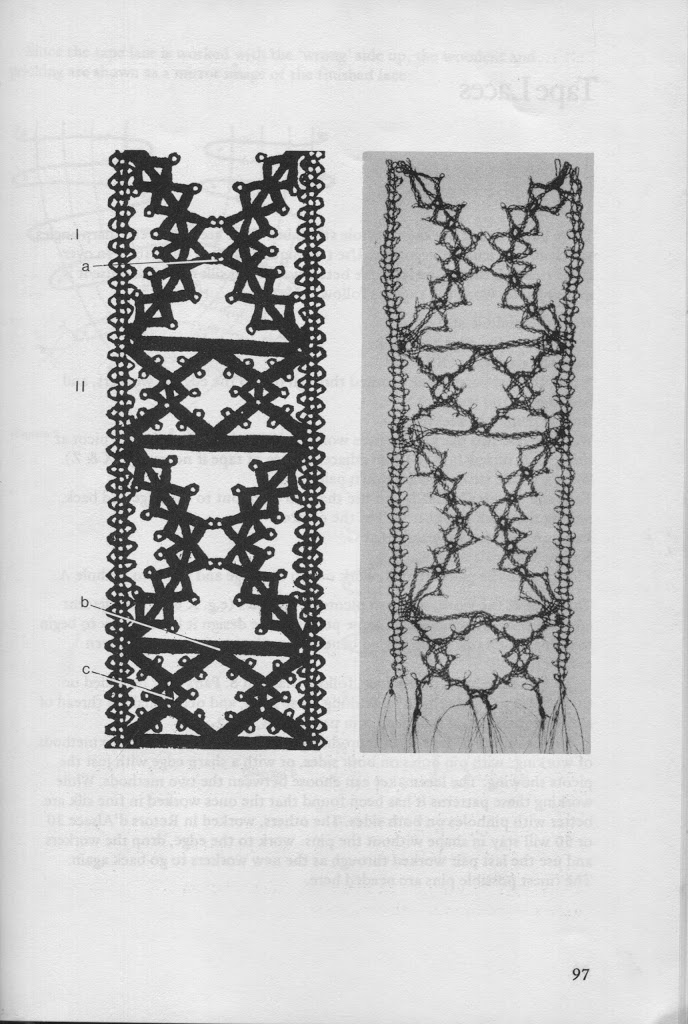This rectangular image appears to be a page from a book, indicated by the number "97" in the bottom right corner. The page features a white background with two vertical strips resembling intricate ribbons or embroidered patterns. These strips are very similar, sharing the same design, yet differ in their presentation. The left strip is a detailed illustration of the pattern, complete with black zigzag designs and various ornate knots. It includes several letters such as A, B, C, H, and L, along with arrows pointing to different sections, suggesting a step-by-step instructional guide. The right strip seems to represent the finished product or perhaps the back side of the ribbon, presented in shades of gray with the designs appearing less bold. There are faint outlines of text from the opposite page visible through the paper, though they are too faint to be read. Overall, the image captures a study of detailed pattern work, likely demonstrating a form of traditional knot tying or embroidery.